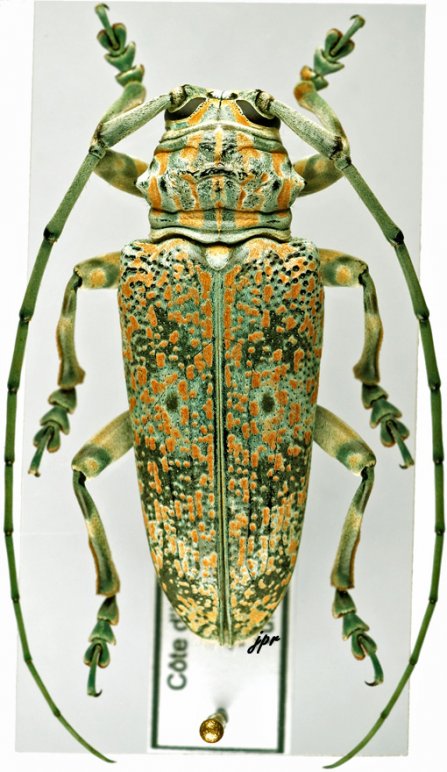The image features a highly detailed and colorful beetle-like bug, showcased in what appears to be a museum exhibit on a light gray slide with a white and green label at the bottom, secured by a gold pin. The bug predominantly displays vibrant green and yellow colors, with yellow and orange spots scattered across its body. Its head is a mix of green and orange with vertical stripes, and it has strikingly long green antennae that extend and curve around its body. The bug possesses six legs: two front legs extending forward from beneath its head, and two pairs of legs attached to its body, stretching backwards. The image is closely cropped, focusing entirely on the intricate details of this vivid insect specimen.